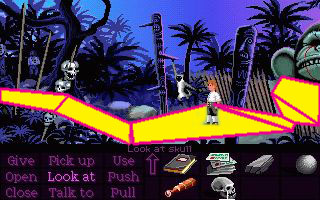This color screenshot from one of the Monkey Island point-and-click adventure computer games features a small, redheaded boy in a white shirt and black pants standing on an oddly sectioned walkway outlined in hot pink and yellow. The background portrays a nighttime jungle scene accented by dark blue and black hues. Silhouettes of palm trees dominate the setting, creating an eerie tropical atmosphere. On the left side of the image, a stake with multiple skulls and a gray spider monkey swinging from a tree branch add to the macabre aesthetic. A partial view of a menacing green monkey's face is visible on the far right. The lower half of the screenshot consists of a black void filled with a menu and several commands in purple text, organized into three columns: "give, open, close," "pick up, look at, talk to," and "use, push, pull." Adjacent to the menu, there are five item icons: a book, a stack of papers, a stone slab, a dark orb that might be a black ball, a spyglass, and a skull. The image is slightly wider than it is tall and evokes a strong sense of classic pixel art from early PC games.